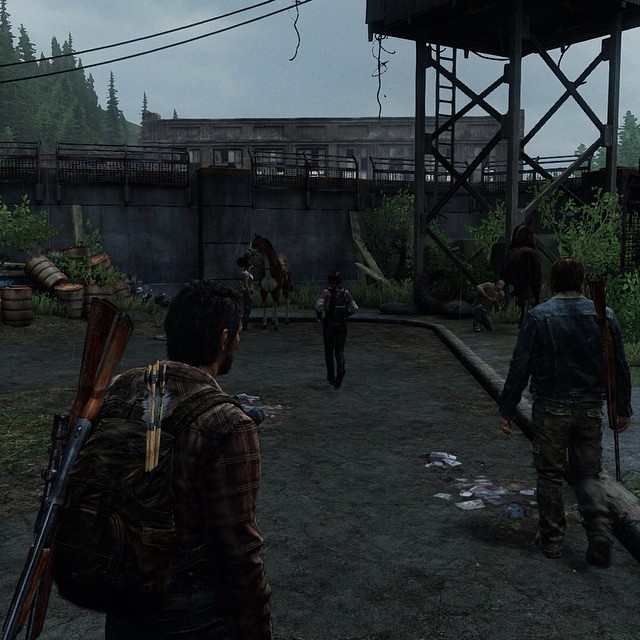This is a color screenshot from a dark and atmospheric video game, resembling titles like The Walking Dead or The Last of Us, with a grim, apocalyptic setting. The scene captures an outdoor environment under a dim sky, hinting at an oppressive, brooding atmosphere. In the foreground, a character, wearing a striped shirt, carries a rifle and a bow with arrows on his back, while three other characters, two of who are visibly armed and dressed similarly in dark, rugged attire, walk ahead along a shadowy path. The ground is littered with debris, enhancing the desolate vibe.

In the background, you can discern faint images of a concrete wall topped with a fence and a large water tower with a steel, circular base, accessible by a visible ladder. There are also dark silhouettes of evergreen trees and power lines in the distance, with the entire scene being shrouded in shadows, making it look almost indistinguishable at parts. The presence of both natural and man-made structures, with the gloomy setting and scattered garbage, paints a bleak picture of survival in a post-apocalyptic world.